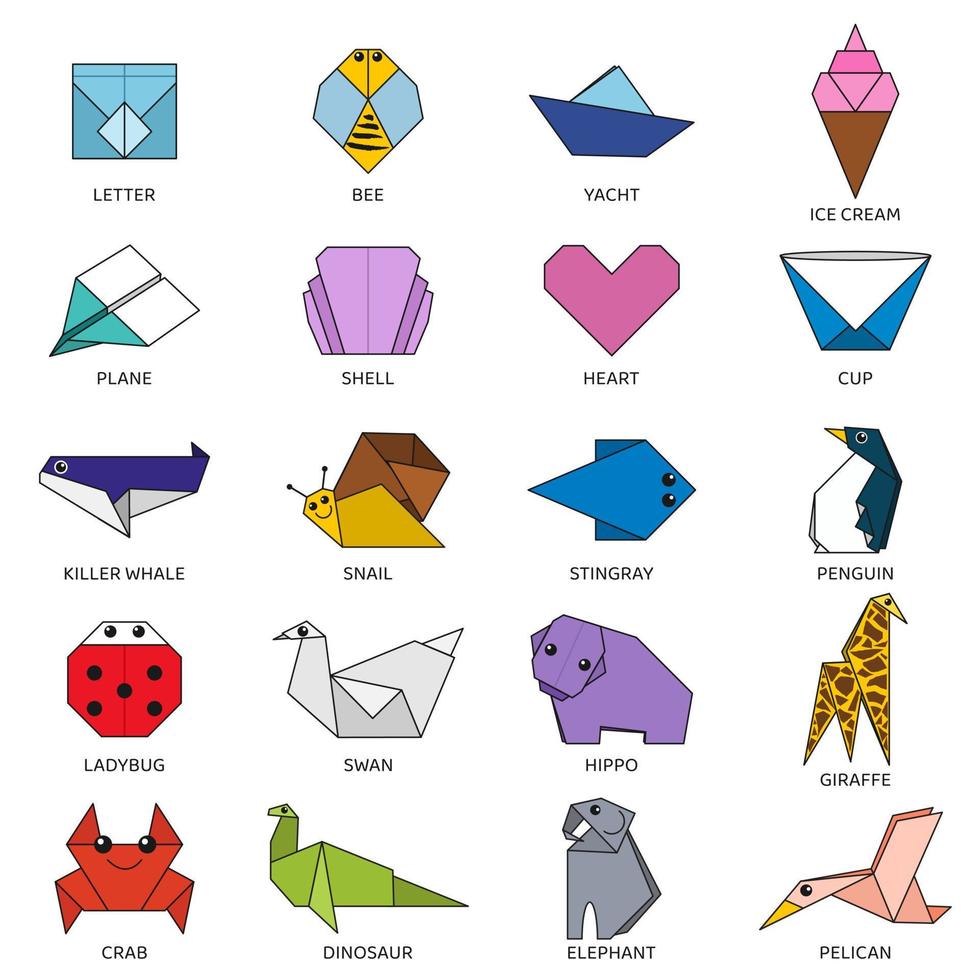This image features a detailed and colorful arrangement of 20 origami illustrations, each showcasing a different object. The objects are neatly organized into five rows and four columns, against a plain white background. Each origami creation is outlined in black and filled with vibrant colors, and all are labeled with their respective names beneath them. 

From left to right, the top row includes a blue envelope letter, a blue and yellow bee, a blue and light blue yacht, and a brown and pink ice cream cone. The second row features a paper airplane, a purple seashell, a red heart, and a white and blue paper cup. The third row showcases a blue and white killer whale, a yellow snail, a blue stingray, and a white and black penguin with a yellow beak. The fourth row displays a red, black, and white ladybug, a white swan, a purple hippo, and a giraffe made from patterned yellow and brown origami paper. Finally, the fifth row includes a red crab, a green dinosaur, a gray elephant, and a pink pelican with a yellow beak. 

Overall, the image serves as a visual guide to the various items one can create through the art of origami.